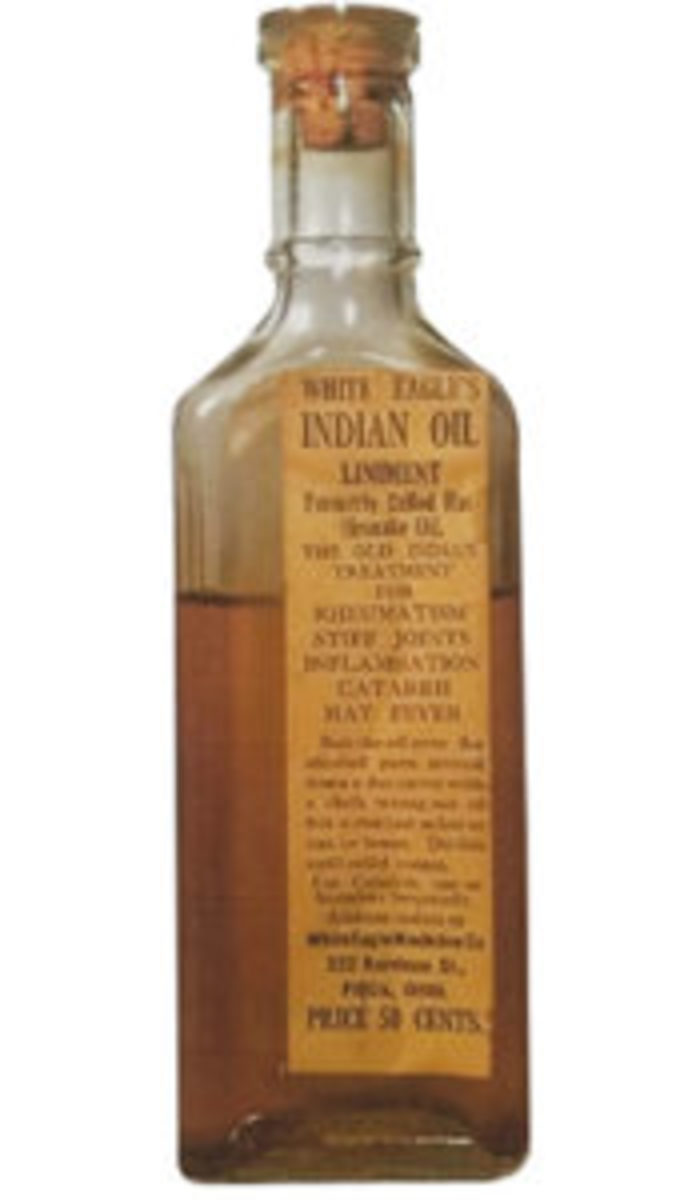This photo features a small, vintage glass bottle filled approximately three-fifths to three-quarters full with a dark, brownish-yellow oil, presumed to be liniment. The bottle has a rectangular shape with a corkscrew top securely in place, suggesting its age and the era it hails from. The label, aged and stained to a yellow-brown hue, prominently reads "White Eagles Indian Oil Ointment," though the rest of the text is largely illegible due to blurriness. At the bottom of the label, the price is clearly marked as 50 cents. Despite the label's weathered condition, it hints at the historical and possibly medicinal nature of the contents.